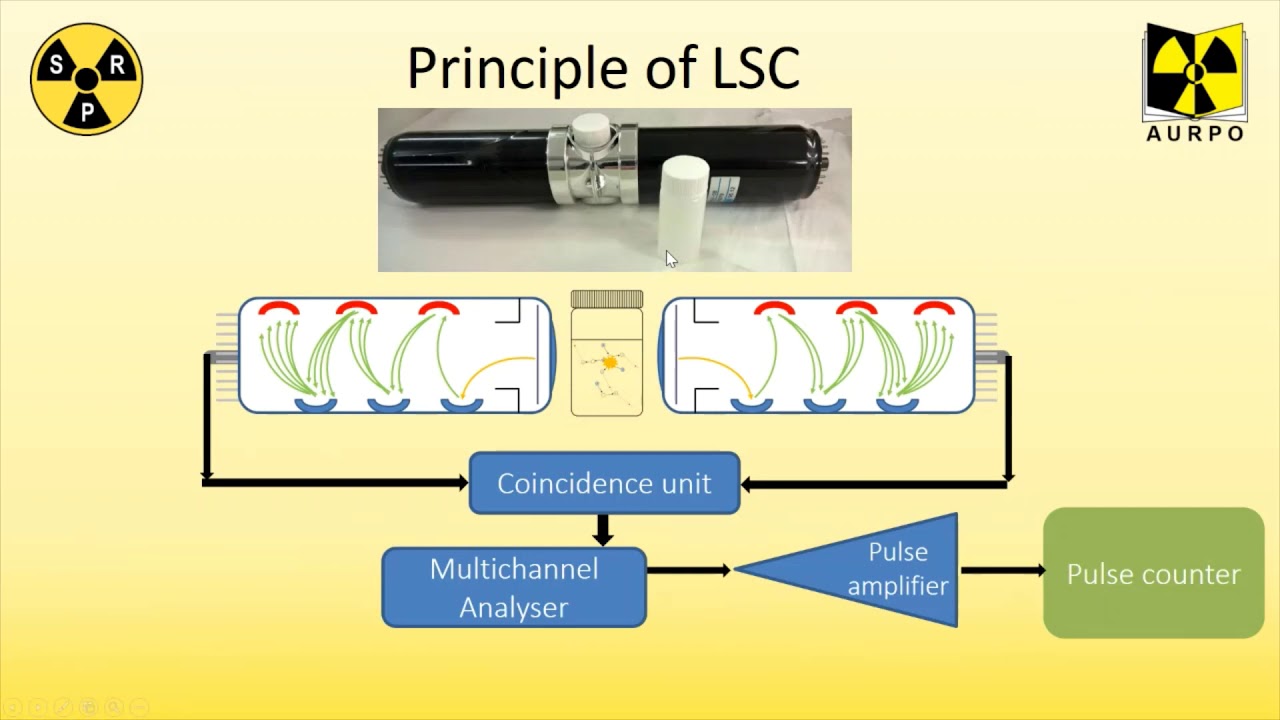The image is a detailed page from an instruction manual, complete with a section titled "Principle of LSC" prominently displayed at the top center. The page features a peach-to-yellow gradiated background, and includes both a photograph and a diagram of the object in question. The photograph, appearing in a small rectangle at the top, shows a black object with a white button, while the flow chart below outlines the unit's functioning. This flow chart begins with the "Coincidence Unit," transitions to the "Multi-Channel Analyzer," and then splits off into the "Pulse Amplifier" and "Pulse Counter." In the upper left-hand corner, a yellow circle housing three black triangles each marked with the initials "S," "R," and "P" (forming a radiation symbol) is present. In the right-hand corner, there's a drawing of a book, with the letters "AURPO" printed beneath it. The thorough explanation and clear labeling suggest that the manual is designed for someone knowledgeable in the field.